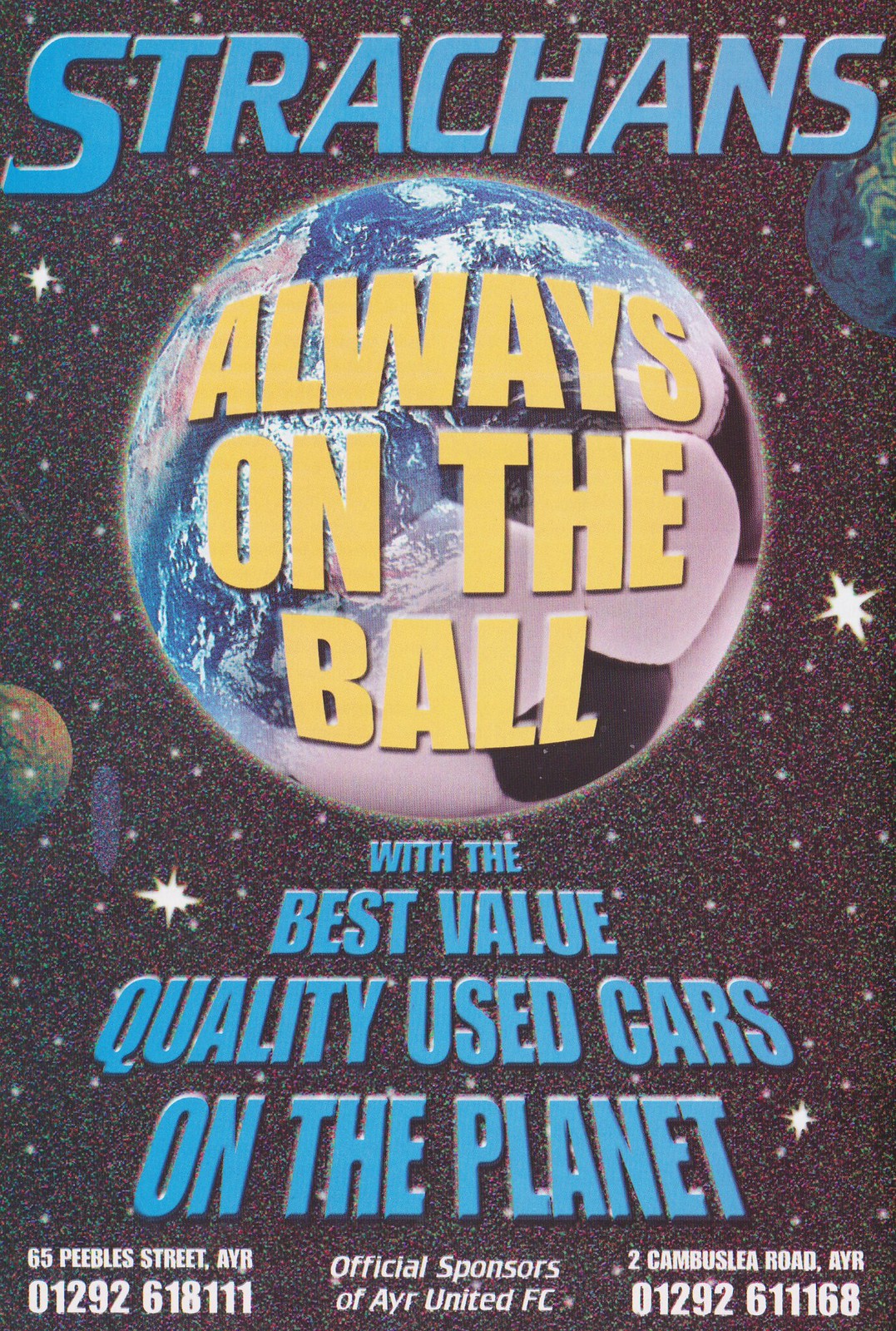This advertisement for Strachans, set against a star-studded space backdrop, features a captivating central image of a soccer ball merged seamlessly with the Earth. The top of the ad showcases the large blue text "Strachans," while the slogan "Always on the Ball" arcs gracefully across the ball/globe in bold yellow letters. Below, additional blue text highlights the dealership's promise: "With the best value quality used cars on the planet." At the bottom, the ad lists two addresses: "65 Pebble Street, ABR, 01292 618111" on the left and "2 Cambuslia Road, AYR, 01292 611168" on the right. Central to the addresses, the ad proudly states, "Official sponsors of Ayr United FC." The design integrates smaller planets and stars, enhancing the cosmic theme.